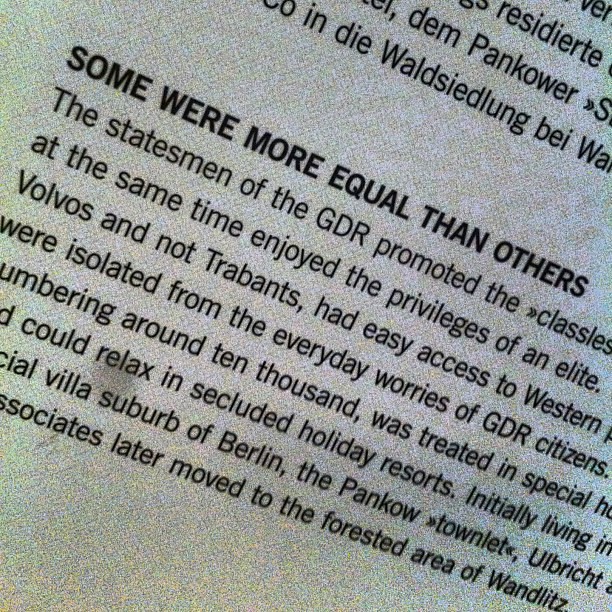The image is a close-up of text that appears to be from a book, a newspaper, or possibly a magazine. The text is oriented sideways, with the beginning at the top left and the end at the bottom right. The background is off-white, and the text is in bold black font. The prominent header reads in all caps: "SOME WERE MORE EQUAL THAN OTHERS." Below this, smaller black text presents a partly cropped narrative about the statesmen of the GDR. It discusses how these leaders, who promoted classlessness, simultaneously enjoyed elite privileges. They had access to Volvos and Trabants, were shielded from the daily struggles of GDR citizens, and lived in privileged conditions. The text mentions their seclusion in holiday resorts, residence in the villa suburbs of Berlin, particularly Pankow, and later relocation to the forested area of Wanditz. The grainy quality of the image suggests it may be a photograph taken with a low-resolution camera, and parts of the text are cut off, making it difficult to fully decipher the entire passage.